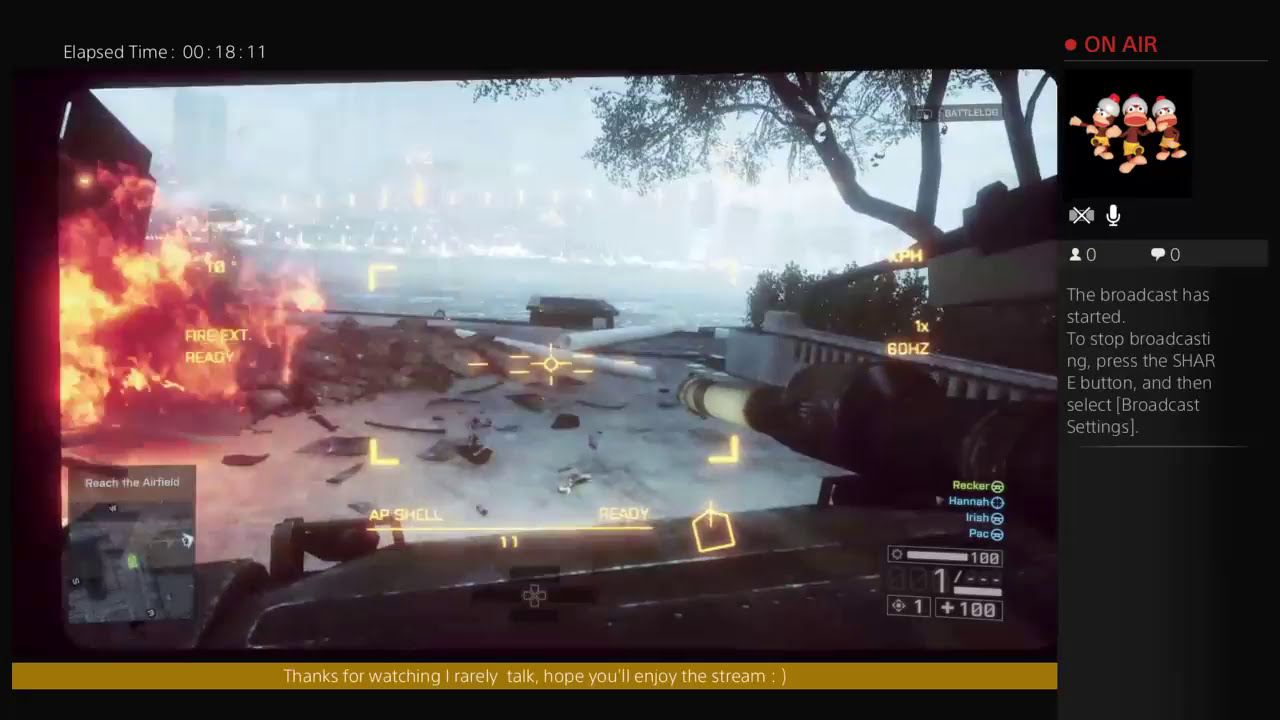This image is a screenshot from a live stream of a video game. The elapsed time of the broadcast is 00:18:11, located in white print at the upper left corner. The top right corner shows a red dot accompanied by the text "on air" in red letters, signifying that the stream is live. The main scene of the game depicts a tank in the forefront, actively engaged in combat with explosions and fire evident on the left-hand side. The backdrop includes a gray landscape with rubble, a tree on the right side, a railing, and a body of water that separates the tank from a cityscape in the distance.

Three brown monkeys with red mouths and white caps featuring red details are seen in a black square block beneath the elapsed time. Below them, there’s a microphone icon and other icons indicating stream interactivity, such as a head-and-shoulders figure, a messaging bubble, both marked with zeroes. Additionally, there’s text indicating that the broadcast has started, followed by instructions to stop the broadcast by pressing the share button and selecting broadcast settings.

At the bottom left, a banner with white text on a black background informs viewers, "Thanks for watching. I rarely talk. Hope you'll enjoy the stream." Overlaying the game scene, more text in white on gray denotes game objectives, such as "Reach the airfield." The chaotic battlefield is characterized by concrete debris from explosions, further emphasized by intermittent gameplay text like "Fire next ready."

In the overall setting, various UI elements from the game and streaming platform emphasize the live nature of the broadcast and provide additional context, such as health status, player names, and stream engagement metrics. The scene encapsulates a live gaming session amidst an intense and destructively vibrant virtual environment.